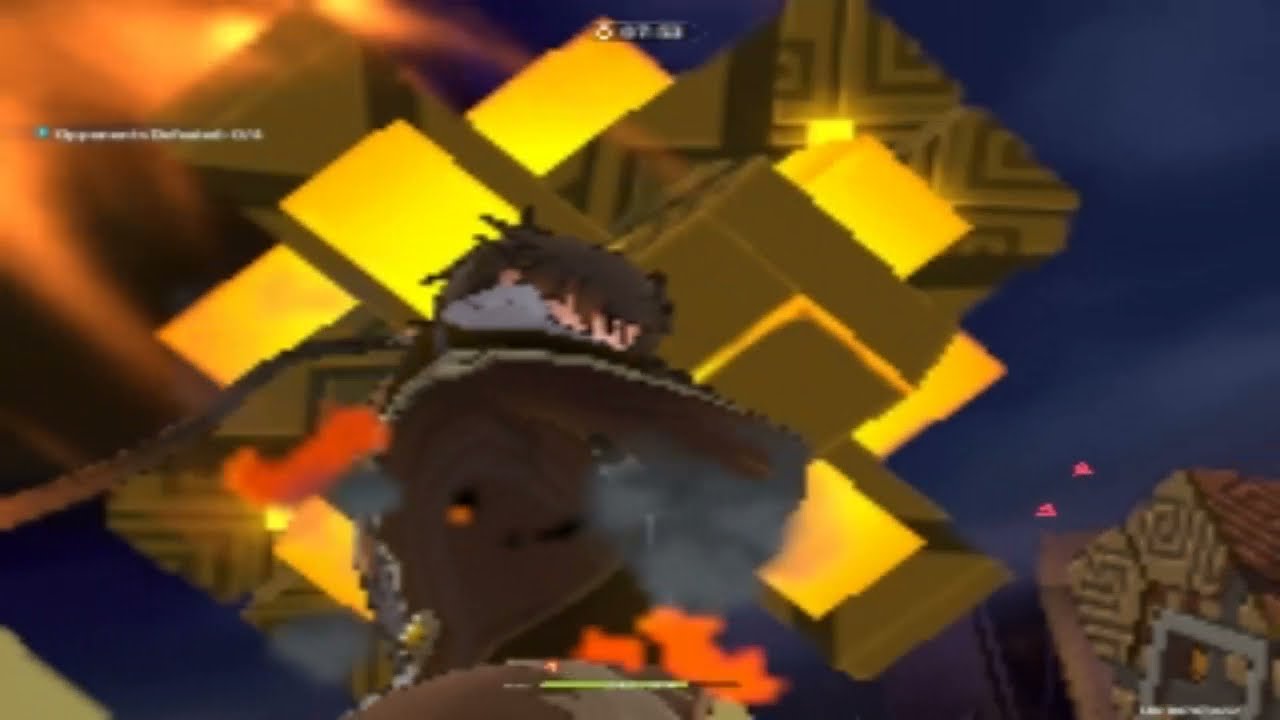The image appears to be a screen grab from a video game predominantly featuring a blue-toned sky with small, barely visible white clouds. Central to the image is a male character with dark, short brown hair partially covering his face, giving the impression of a samurai figure in a brown robe or jacket with a large hood. His right arm appears to be raised, possibly to shield his identity or protect himself. Bright orange light swirls behind him, resembling rocket exhaust or flames.

A gold rectangular box with geometric shapes and intricate black swirls is positioned in the bottom right-hand corner, bearing a large gray square on its surface. Directly behind the character is a large, floating golden object similar in pattern to the box, potentially indicating a spaceship or machine. Scattered across the scene are several yellow rectangles or squares arranged diagonally on different parts of the screen, some set against dark blue and brown backgrounds.

In the upper left corner, a glowing orange flare is visible alongside a small, unreadable gray text bar. Indistinct icons, including a possible health meter, are located in the top center. On the right side of the character are two red, triangular target markers, adding to the gaming interface’s complexity. The bottom-left section features a diagonal blue bar matching the background’s hue. Together, these elements create a dynamic, albeit somewhat abstract, composite of shapes and forms intrinsic to the video game environment.